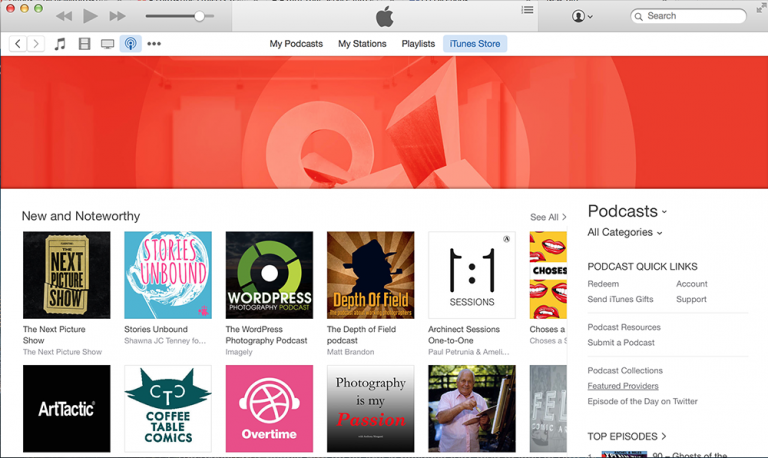This is a detailed descriptive caption for a computer screenshot:

The screenshot captures the interface of a media application. At the top of the screen is a horizontal gray rectangle functioning as a control bar. In the upper left corner of this bar are three small circles—red, orange, and green—aligned horizontally. To the right of these circles, the control bar includes media control buttons: double left-pointing arrows for rewind, a single right-pointing arrow for play, and double right-pointing arrows for fast forward. Adjacent to these buttons is a slider with a movable white circle indicating the track's position.

Centrally located within the control bar is the Apple logo. On the right side of the bar, there is a profile icon featuring a circle with a down arrow next to it. Further to the right is an elongated white search bar with a magnifying glass icon and the word "Search" inside it.

Beneath this control bar is a menu bar offering various navigational options. Directly below the menu bar is a prominent red rectangle with a design element that resembles a white "O" and a number "1", though the bottom part appears to be cut off despite being intact.

In the section below the red rectangle, the left side displays bolded black text reading "New and Noteworthy." Adjacent to this text are six squares arranged horizontally, though only the left half of the sixth square is visible. The first square prominently features the cover for "The Next Picture Show," indicating a collection of 12 images.

On the right side of the screenshot, there is a list titled "Podcasts," showcasing a selection of available podcast options.